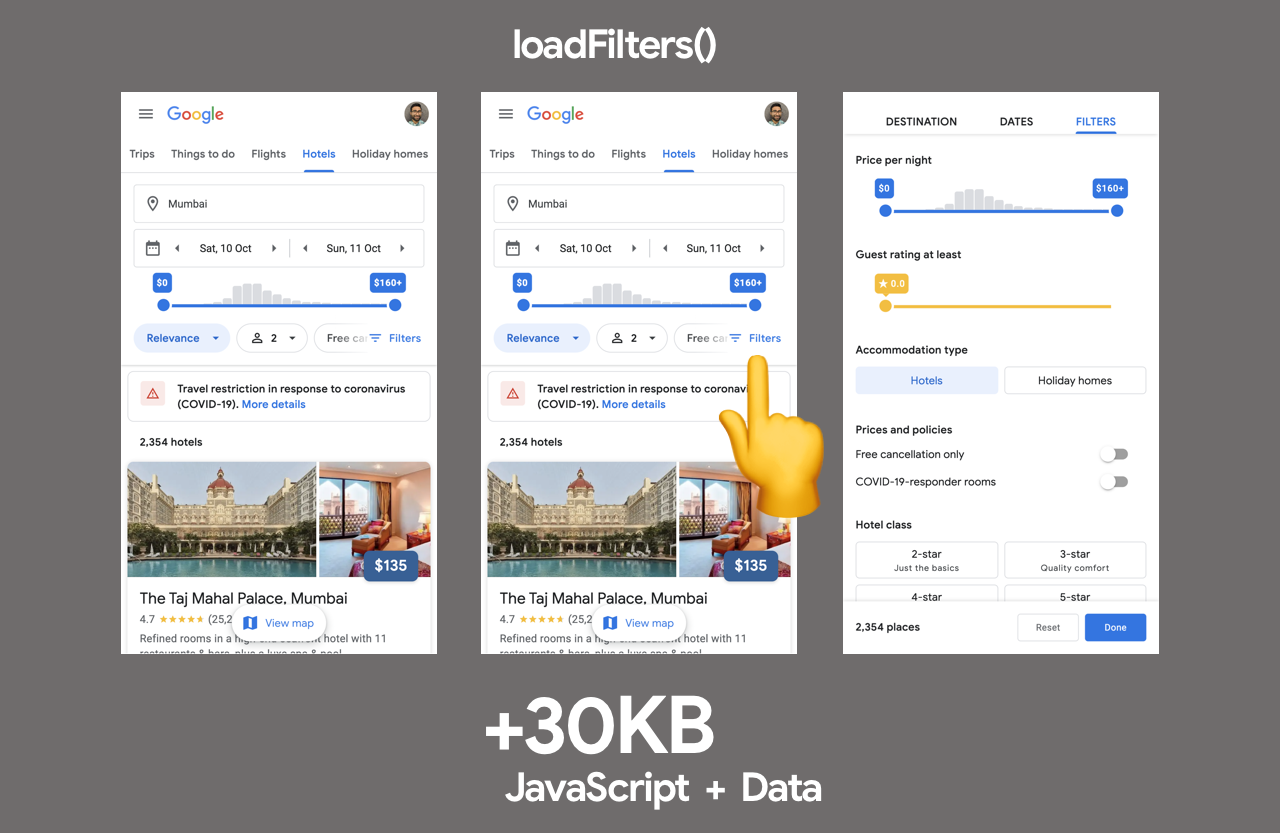This compositional image consists of two juxtaposed screenshots from a Google search results page focusing on flight plans and travel information. 

On the left screenshot, prominently displayed is the Google search interface with a top banner featuring the Google logo and links for "Trips," "Things to do," "Flights," "Hotels," and "Holiday homes." Below this, there's an indication related to travel restrictions due to coronavirus (COVID-19) with a "More details" link. Distinctly visible in this screenshot are references to the iconic Taj Mahal Palace in Mumbai.

Moving to the right screenshot, there is a close-up showcasing a hand pointing towards the "Filters" option on the flight search interface. Below this interactive element, options for specifying destination, dates, and applying filters are apparent. The visible price filter ranges from $0 to $160+.

The color scheme across both images prominently includes shades of blue, white, and red. The background of the composition is predominantly gray. Annotations at the bottom note the image file size, which exceeds 30 kilobytes, and mentions that JavaScript elements and data contribute to its composition.

Overall, this detailed visual representation provides a snapshot of user interactions on Google while seeking flight information, underscoring the available filters, options, and travel advisories.